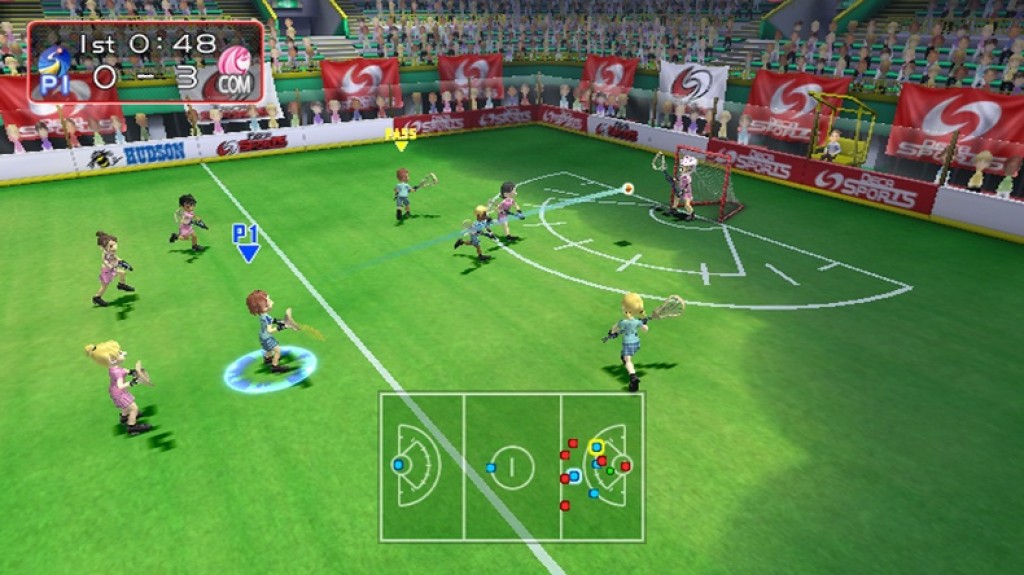The image depicts a scene from a computer game set in a vibrant, virtual stadium. At the top left corner, digital text indicates "First, 0:48" in white, suggesting 48 seconds into the first period of play. The score reads "0 to 3" with a blue helmet icon labeled "P1" on one side and a pink helmet labeled "COM" on the other. The game takes place on a lush green field surrounded by a packed audience in the stadium stands. Approximately ten players are visible on the field, engaged in intense action. Prominently featured is a football goalpost, where a ball is being thrown and a goalkeeper is poised to block it. The scene captures the dynamic and immersive atmosphere of the game, emphasizing the competitive spirit and detailed visual environment.